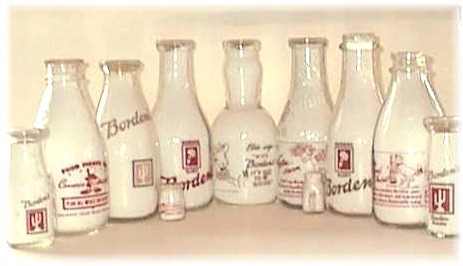The image features a collection of vintage or commemorative Borden milk bottles displayed against an off-white background and atop a matching surface, likely a photographic drape. The lineup includes around ten bottles in various sizes and shapes, arranged from smaller bottles on the left, to taller ones in the center, and smaller ones again to the right. Most bottles are filled with milk and have red and black printing, including the name Borden and illustrations of Elsie the Cow. Some of the bottles are capped, and the overall white-on-white composition highlights the antique or commemorative nature of these dairy product containers.